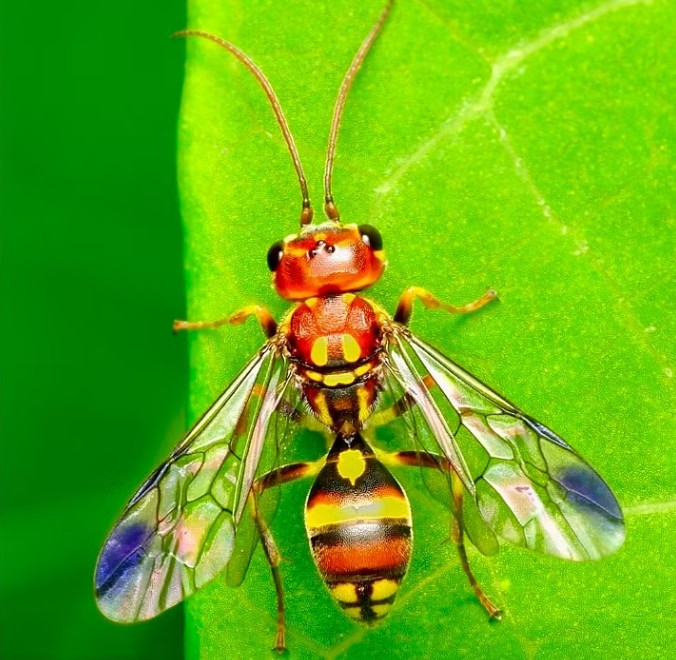This high-quality, close-up photograph features a detailed view of a wasp perched on a vibrant green leaf, showcasing its intricate anatomy and vibrant colors. The wasp, centrally positioned and magnificently zoomed in, displays prominent yellow, orange, and black stripes on its back, with additional reddish hues on its head. Its transparent wings, adorned with touches of blue, pink, and purple at the tips, reveal dark veins coursing through them. The wasp's large, bulging black eyes flank its head, which sports long, segmented antennae. The leaf beneath the wasp is equally detailed, with visible veins and a slight yellow tint, possibly sprinkled with pollen. Remarkably, the wasp’s thorax features yellow spots that form an almost happy face pattern, further adding to the visual intrigue of this striking image.